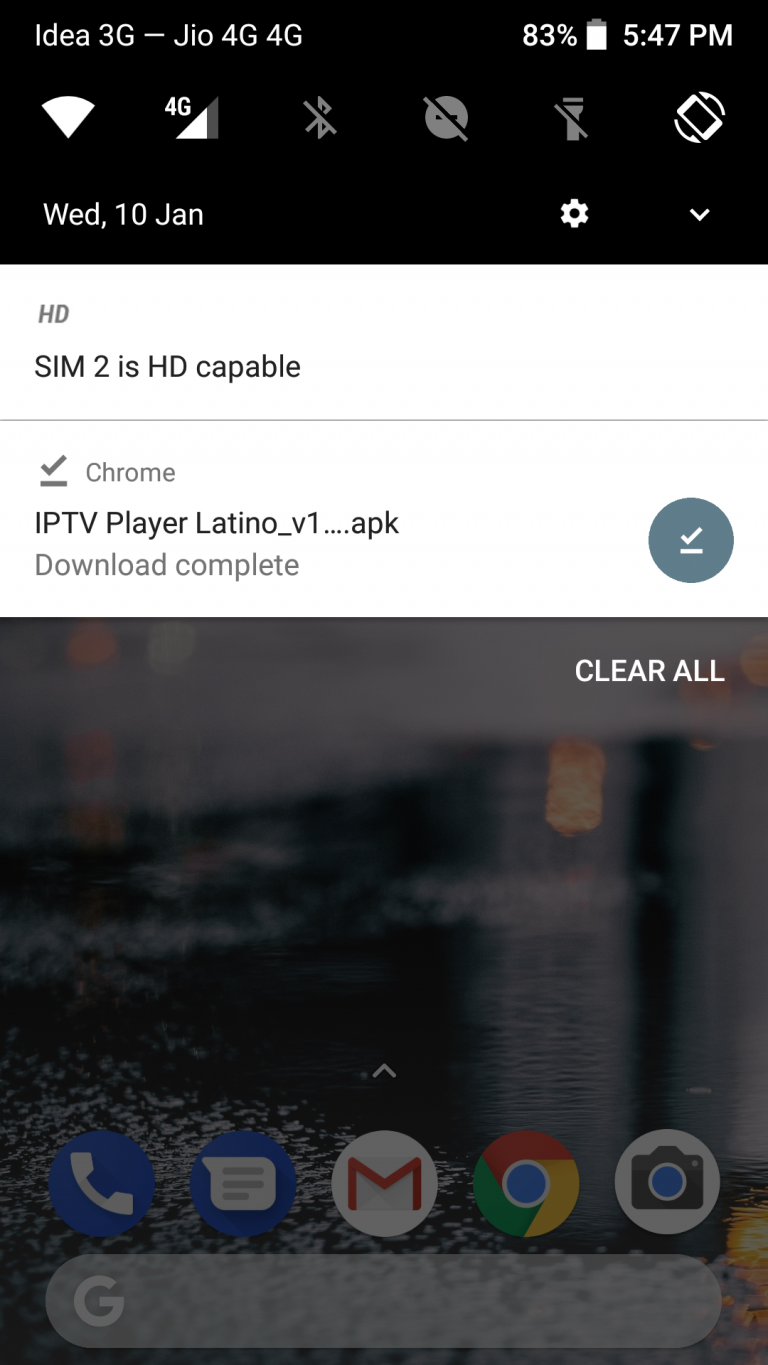The image appears to be a screenshot taken on a smartphone, displaying various status icons and notifications. At the very top, a black status bar features multiple indicators. On the left, "IDEA3G-JIO4G4G" is displayed in white text. Moving right, a battery icon shows a charge of 83%, followed by the time, "5:47 PM." Further to the right, an upside-down white triangle is visible, next to a "4G" icon with a partially filled white triangle. Additional symbols include a zigzag line with a slash through it, a circle with dots and a line through it, and a flashlight icon with a line through it, as well as a phone icon with arrows pointing up and down.

Below this, the screen displays the date as "Wednesday, 10 January," accompanied by a gear icon on the right. Underneath, a white section reads "HD SIM2 is HD capable," separated by a gray line. Another white area follows, stating "✓ Chrome. IPTV player Latino_V1... APK download complete." At the bottom, a large gray square contains the option to "Clear all."

The bottom of the screen shows a row of app icons: a phone (call) app, messaging app, email app, Chrome browser, and a photos app. Above these icons is a search bar featuring a "G" logo, indicative of Google Search.